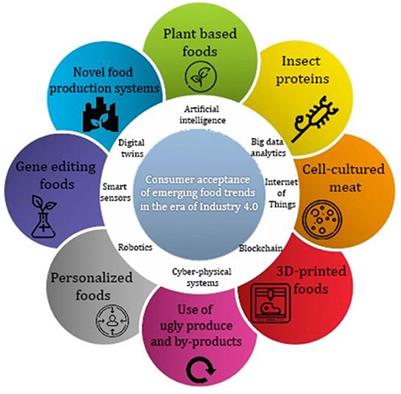The image features a detailed and colorful chart demonstrating consumer acceptance of emerging food trends in the era of Industry 4.0. At its core, surrounded by a gray center circle and a white ring, are terms such as artificial intelligence, big data analytics, internet of things, blockchain, cyber-physical systems, robotics, smart sensors, and digital twins, reflecting the technological influences on food production. Radiating from the center, the chart is divided into various colored segments—each depicting different food categories with corresponding cartoony illustrations. These categories include green for plant-based foods, yellow for insect proteins, orange for cell-cultured meats, red for 3D-printed foods, pink for the use of ugly produce and by-products, gray for personalized foods, purplish-blue for gene-edited foods, and blue for novel food production systems. This visually appealing diagram captures the intersection of high-tech advancements and innovative food sources, providing insights into public acceptance of these new food trends.